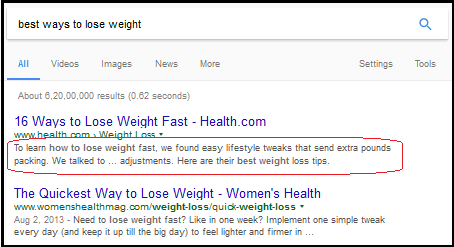This image depicts a Google search results page with a query for "best ways to lose weight." The search bar at the top, featuring the query in black text against a white background, is prominently displayed. Just below, a light gray navigation menu presents options for "All," "Videos," "Images," "More," "Settings," and "Tools." A brief summary below the menu indicates that approximately six million results were found in 0.62 seconds.

The search results begin with a prominent listing from Health.com titled "16 Ways to Lose Weight Fast." This entry's website URL is displayed in green text beneath the title, followed by a brief snippet from the article. This specific result is highlighted with a red circle for emphasis.

The second result features another Health.com article titled "The Quickest Way to Lose Weight," with its publication date noted as August 2, 2013. This entry also displays the URL in green and includes a brief excerpt of the article. The entire search results page is framed by a black border, drawing attention to this specific screenshot.